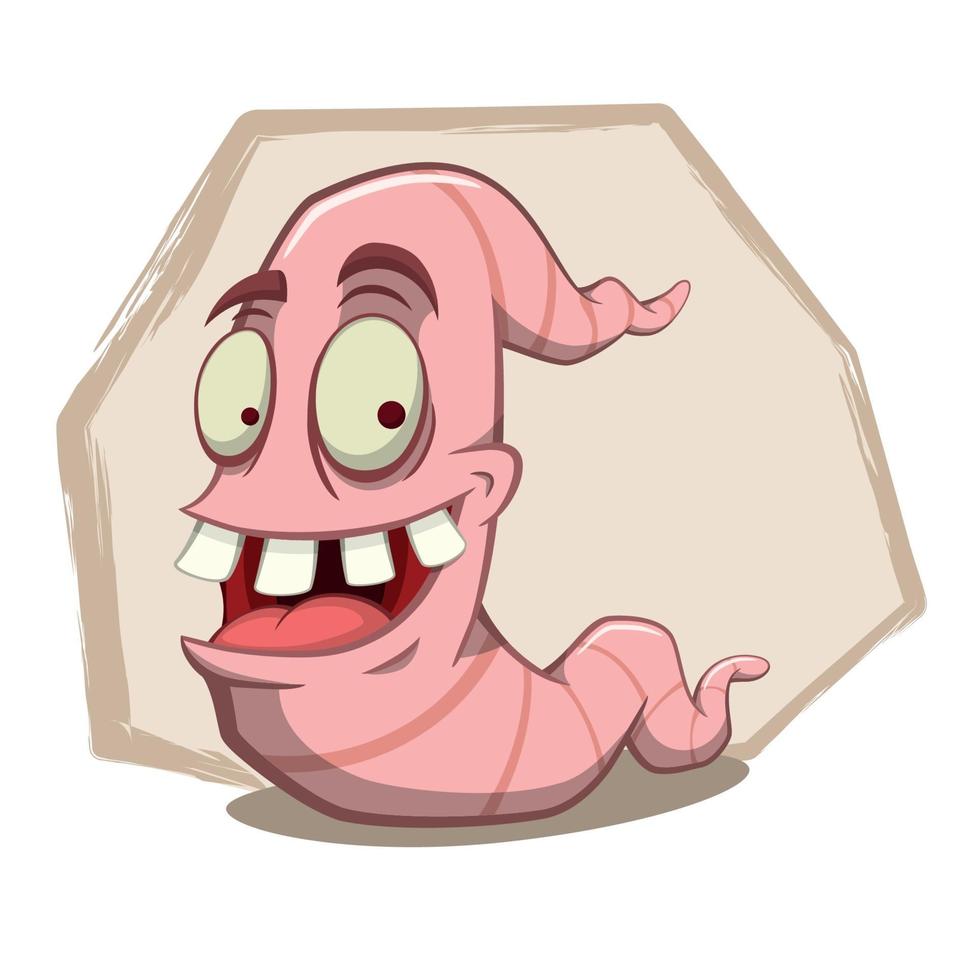The image is a lively, cartoony drawing of a cheerful worm characterized by its distinctive features and vibrant colors. The worm, predominantly pink with darker pink stripes, extends into the background, creating a sense of depth. Its head is particularly notable, boasting an oversized human-like face with wide-open, slightly yellowish eyes, and brown raised eyebrows. The worm's large, buck-toothed grin is accentuated by four prominent teeth on the top, widely spaced, and a big red tongue visible inside its open mouth. Adding to its whimsical appearance, the worm has what seems like a secondary tail or hat-like appendage on top of its head, extending its playful design. The background features a large, tannish-brown hexagonal shape with a darker outline, which provides a contrasting backdrop to the worm’s vivid coloring. Additionally, there's a circular shadow beneath the worm, grounding the character in the scene. Overall, the animated style and detailed depiction of both the worm and its background make the image striking and memorable.